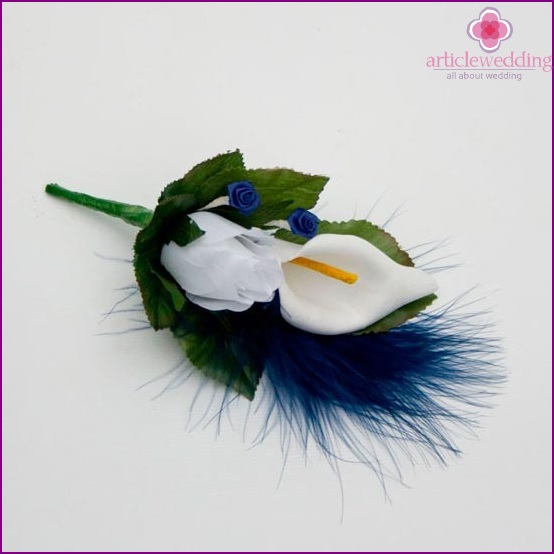The image captures a delicate white-petaled flower with a bright yellow, slender interior where the pollen is typically found. This interior structure is even thinner than the green stem visible at the bottom of the image. Above the main flower, there are striking blue fluffy feathers and intricately crafted blue flowers, which appear to be made of fine, silk-like material. These blue flowers have been skillfully shaped into rose-like forms, demonstrating impressive craftsmanship. Additionally, there are elongated, fuzzy hairs extending from the object, adding to the intricate and whimsical appearance of the composition.